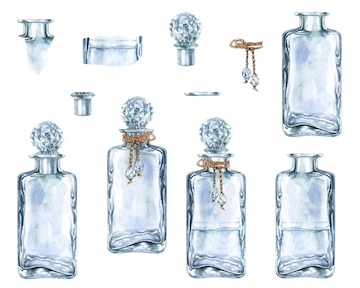The image is a detailed illustration set against a white background, showcasing five silver, white, and gray perfume bottles, resembling decanters, all made of glass. Arranged in two rows, four bottles occupy the bottom row, each with a translucent, rectangular shape. Three of these bottles are capped with crystal ball-like tops, while the fourth bottle remains uncapped. Notably, the two center bottles feature golden chains, akin to bolero ties, adorned with small white crystal beads hanging from the ends, elegantly wrapped around their necks. In the upper row, detailed sketches focus on individual components: a cylindrical crystal cap, a golden tassel, and the bottle neck, all presented separately from the main bottles. The overall composition suggests an advertisement or design study, emphasizing both the intricate accessories and the minimalist, elegant design of the glass containers.